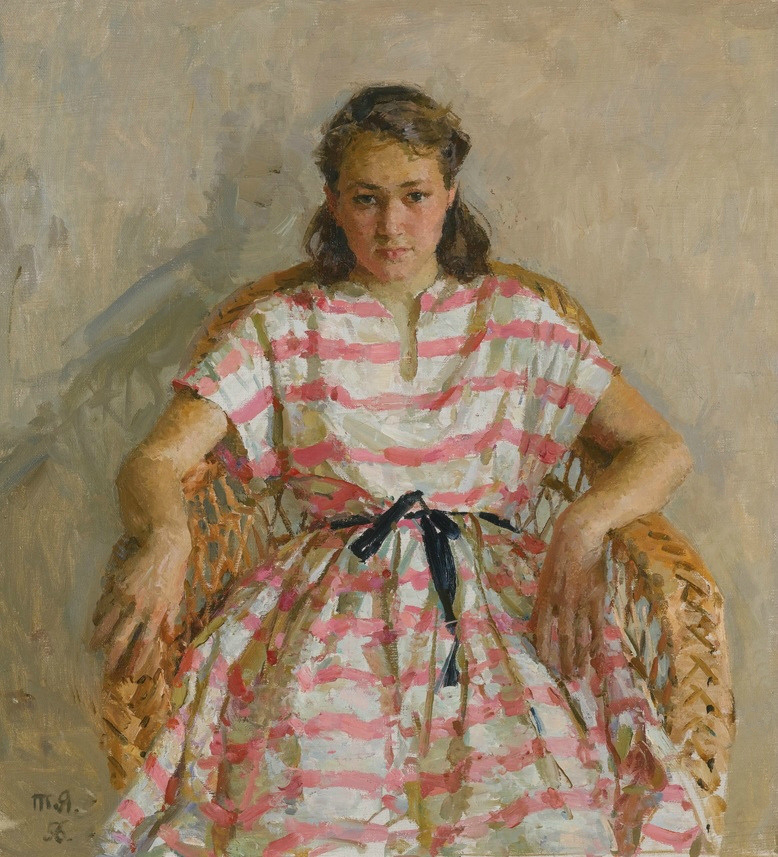This painting, signed "M.A." and dated '56, portrays a young girl or perhaps a young woman, suggesting she is in her late teens or possibly early 20s. She sits in a brown wicker chair against a softly blended background of gray with hints of tan and blue shadows. Her facial expression conveys a sense of mild rebellion or reluctance, as if she has been asked to pose against her will. She gazes directly at the artist with an uninterested, almost defiant stare.

Her hair is a shoulder-length blend of blondish brown, appearing slightly tousled as if she had just come in from the wind. She has large brown eyes that add depth to her emotions. She is dressed in a pink and white striped dress with short sleeves and a modest V-neckline (or slight U-shaped cut), extending beyond her knees, tied at the waist with a black ribbon used as a belt. Her pose is casual, with one arm propped on the armrest of the chair and the other resting in her lap.

The background is an off-white cream color with subtle shadowing, enhancing the focus on her figure. The painting, while not overly detailed, captures her youthful essence and the texture of her surroundings with a charm that evokes the familiar scenes of adolescence and familial obligation.